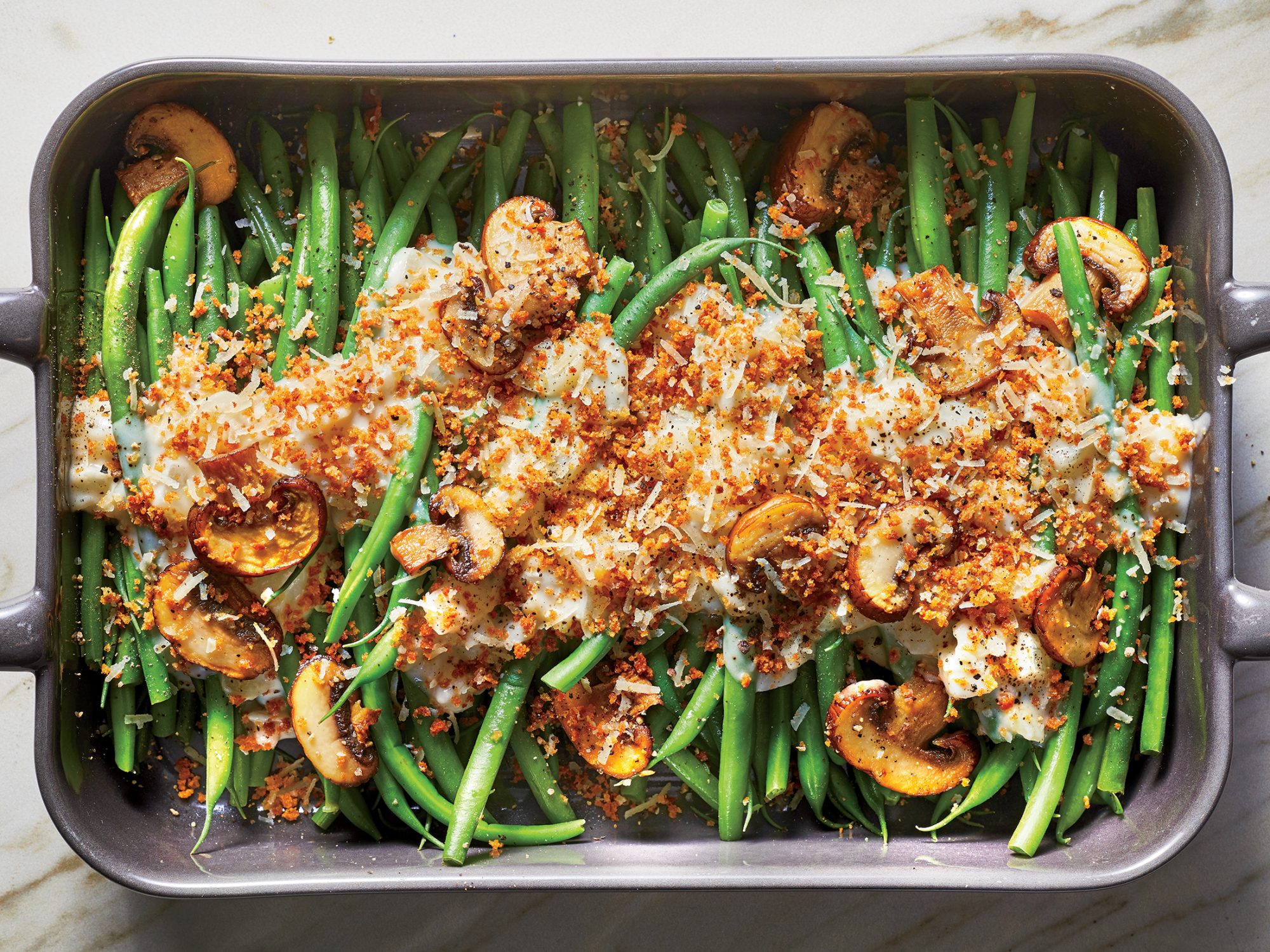The image depicts a top-down view of a baked dish set on a granite countertop with a distinct marbled pattern in shades of white, orange, and brown. The baking dish, made of gray metal with handles on both the left and right sides, contains a generous amount of vibrant green beans arranged vertically. Interspersed among the green beans are sliced mushrooms, browned from the baking process. The dish is topped with a layer of melted cheese and breadcrumbs, which concentrates more in the middle of the dish, leaving the green beans at the edges and corners relatively untouched by the topping. The overall impression is a well-cooked vegetable medley that has been baked to achieve a pleasing golden-brown finish on the cheese and mushrooms.